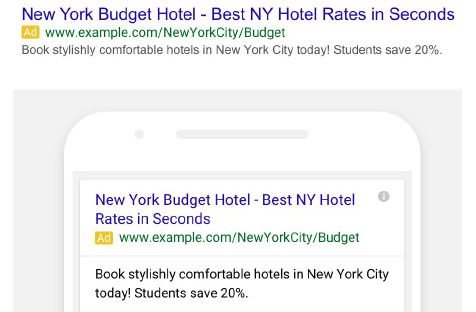Title: Example Search Results for New York Budget Hotels - Desktop and Mobile View

Caption: The image displays two example search results for budget hotels in New York City, highlighting how advertisements appear on both desktop and mobile web browsers. The top half of the image showcases a desktop search result from www.example.com with the headline "New York Budget Hotel - Best New York Hotel Rates," followed by a brief description: "Book stylish, comfortable hotels in New York City today. Students save 20%." The bottom half juxtaposes this with an identical search result designed for mobile browsers, maintaining the same headline, URL, and promotional text. This comparison visually demonstrates how ad placements would appear across different devices, providing insight into the user experience for potential advertisers. These are not real search results but sample representations used for demonstration purposes.